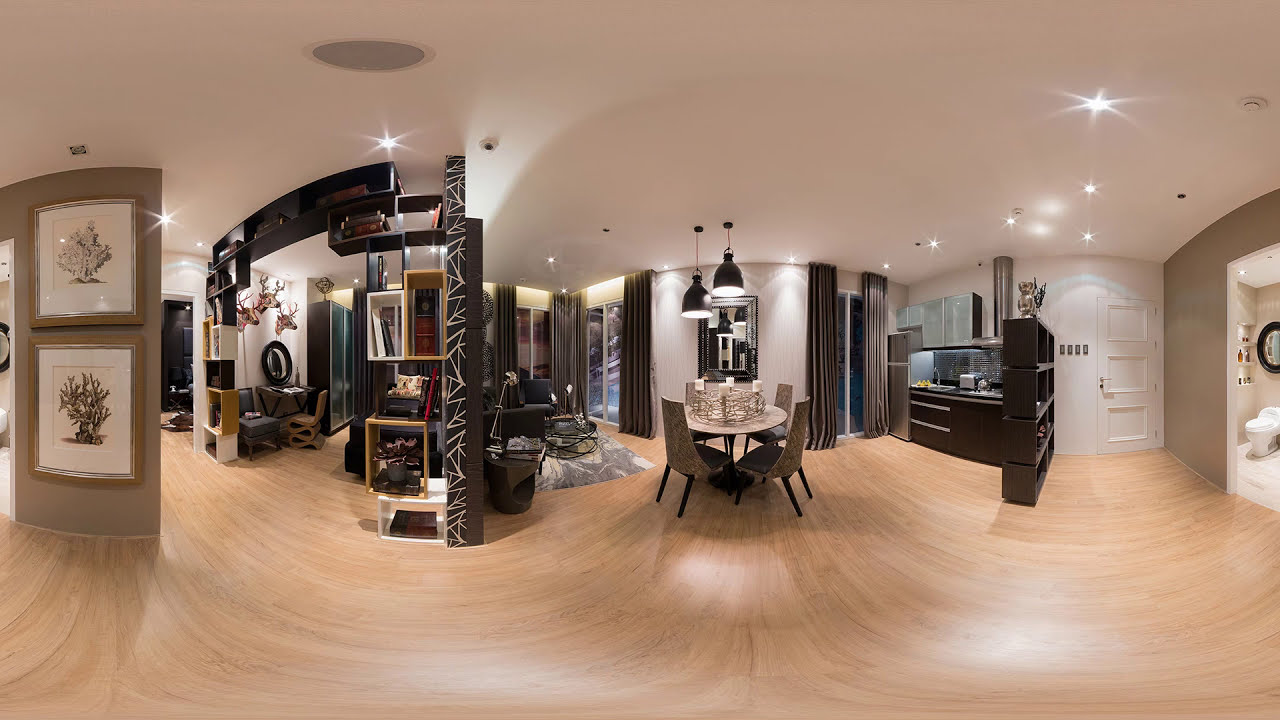The image depicts the interior of a high-end living space or possibly an upscale emporium. The floor is made of luxurious, soft tan wood, which may feature intricate swirls or burl patterns enhancing its elegance. As you enter through the white, multi-paneled front door on the right, you immediately observe a bathroom to the left with a white toilet and a black-framed mirror. The ceiling is entirely white, adorned with spotlights and modern black lanterns, strategically placed to create a star-like illusion indoors.

Directly to the right of the entrance, the space opens up into a sophisticated dining area. The centerpiece is a stylish white circular table surrounded by four tan chairs. Large floor-to-ceiling windows flank the dining table, dressed in dark drapes that frame the natural light beautifully. Behind the dining table, various display cases and bookshelves with individual illuminations showcase an array of decorative items and fine art.

A wall in this space is decorated with framed prints, mostly depicting trees or bushes, set against a darker tan background. There is also a couch positioned on the left side, with a rug spread out in front of it. Adjacent to the couch is a black display with wooden sections showcasing assorted merchandise.

Further into the living space, around the corner, more chairs and shelves are visible. This area has another tan wall adorned with framed prints and modern furniture. The detailed and framed artwork, luxurious flooring, and sophisticated furnishings collectively suggest an upscale, elegant space meticulously designed for comfort and aesthetic appeal.